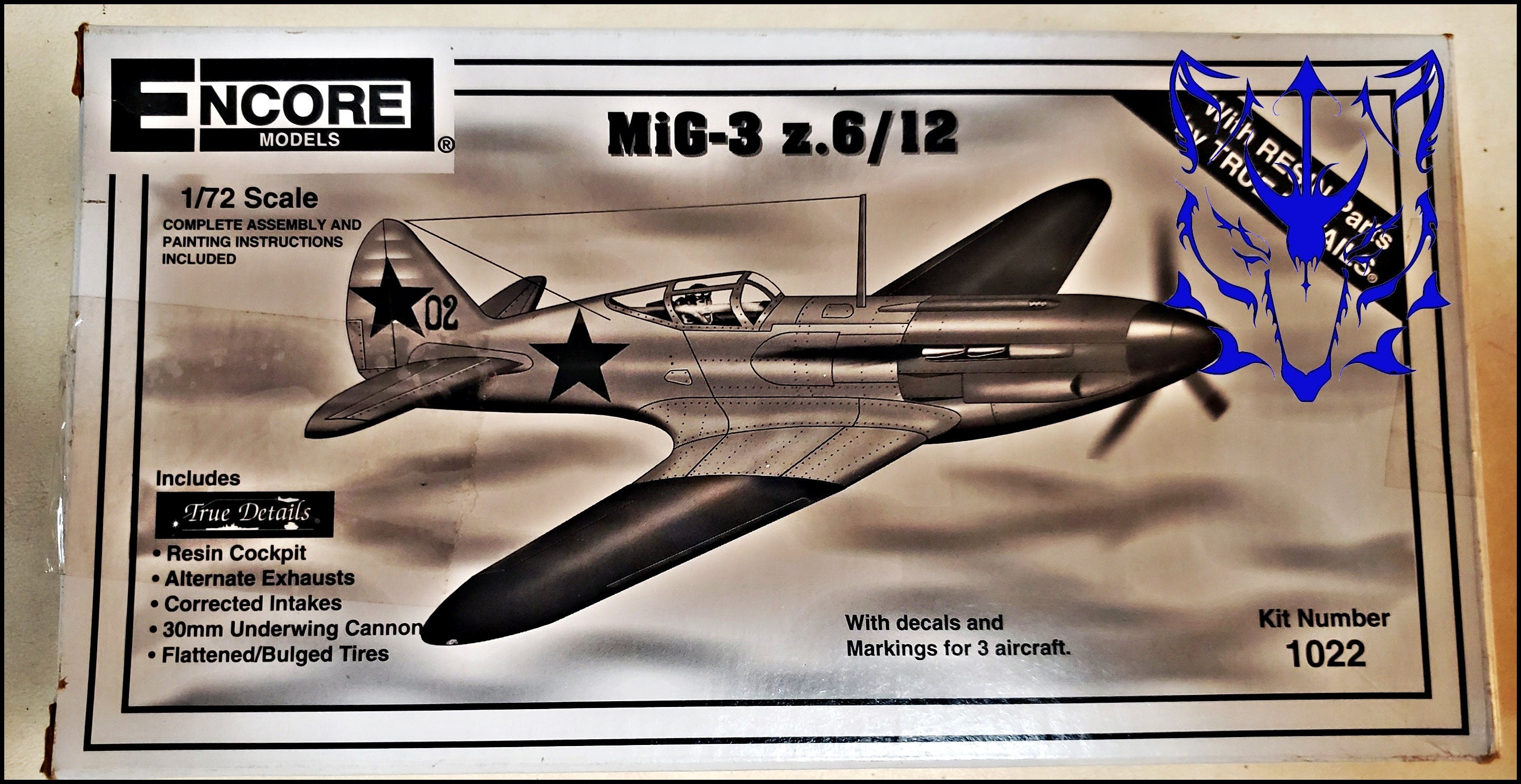The image depicts a detailed box for a model fighter jet, specifically the MiG-3, lying on a surface that appears to be silver. The packaging is predominantly silver with black writing. In the top left corner, the text "Encore Models" is displayed, and at the top center, the model name "MIG-3 Z 6/12" is prominently featured. Along the left side, the scale "1:72" is noted, along with a mention of "complete assembly and painting instructions included." The top right corner features a distinctive blue outline of a wolf, partially overlain by what seems like blue paint splatter. The bottom right corner houses the kit number, "1022."

The central illustration of the MiG-3 model shows a highly detailed aircraft with silvery body and black wingtips. The plane has two large, rounded wings, a propeller at the nose, and visible rivets holding its parts together. The cockpit is covered with clear glass, revealing a pilot inside. Accompanying the artwork are details such as "true details, resin cockpit, alternate exhaust, corrected intakes, 30mm underwing cannon, and flattened bulge tires," and the kit includes "decals and markings for three aircraft." Notably, the aircraft bears two distinctive stars: a black star near the cockpit and another on the tail, which also features the number "02".